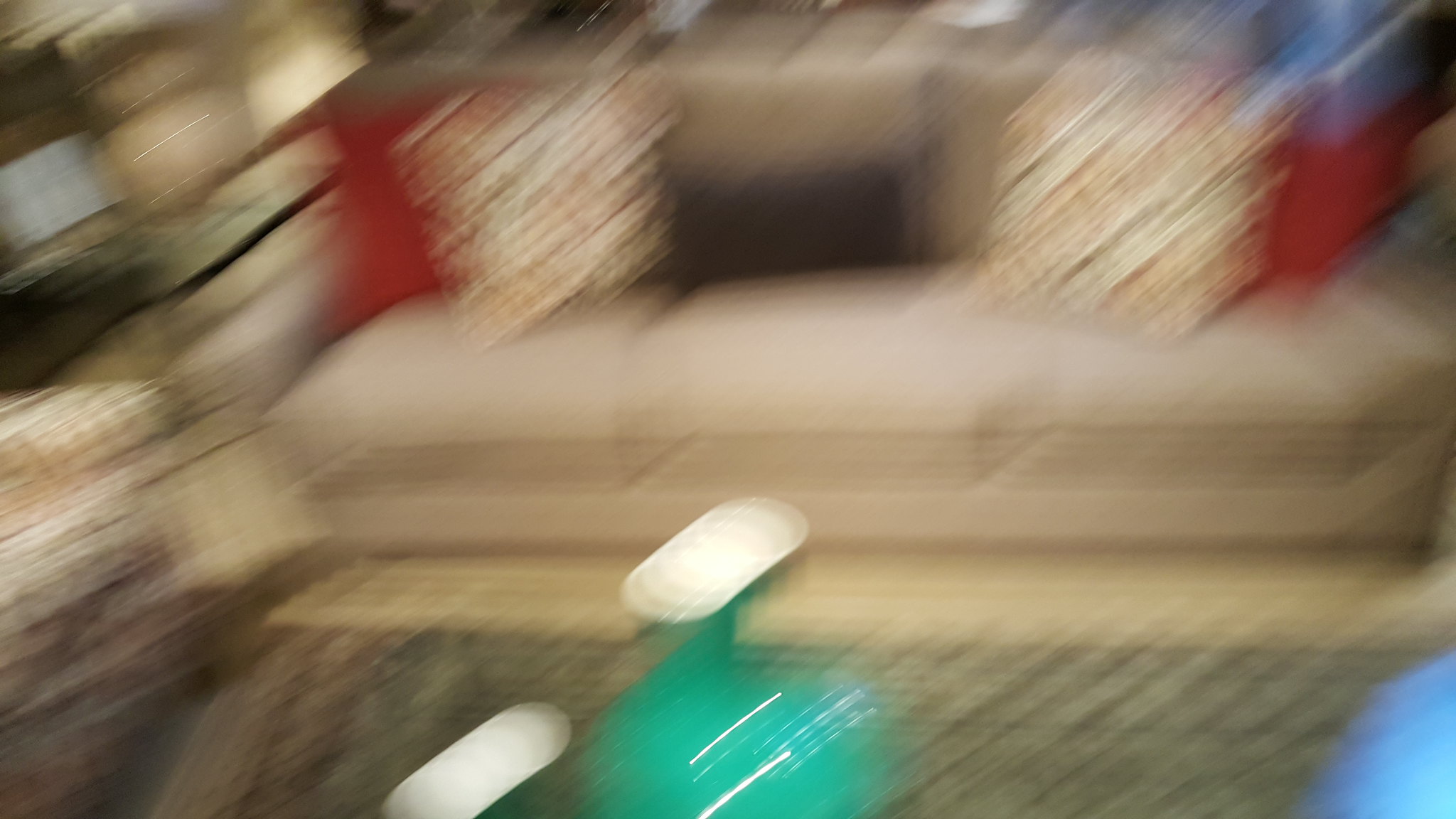This landscape-oriented photograph captures a scene with significant motion blur, suggesting it was taken in a dimly lit indoor environment with the camera in motion. Dominating the image is a beige or tan couch, embellished with an array of throw pillows. The central black pillow stands out amidst an assortment of light yellow and possibly white pillows, with vibrant red pillows bookending the couch on either side. At the lower edge of the frame, two brightly colored objects, likely vases, add to the chaotic yet intriguing composition. Despite the blurriness and streaks of light, the image conveys a cozy, albeit indistinct, setting.